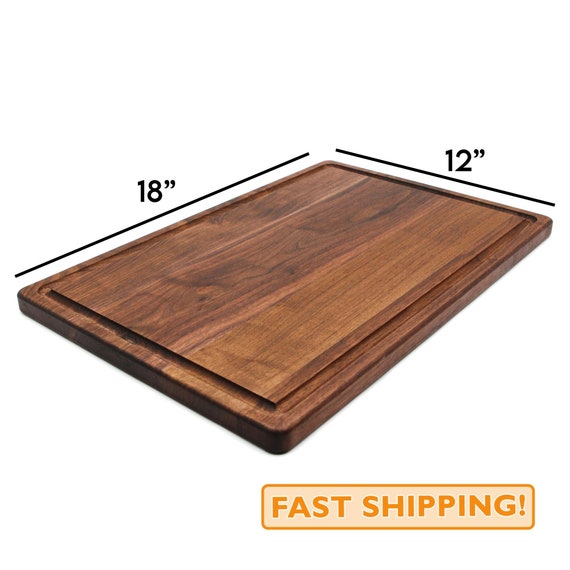The image features a high-quality, rectangular cutting board made from dark walnut wood. The board is shown at an angled perspective, enhancing its dynamic presentation against a white background. The finely grained wood displays a rich, dark brown color with marbling that ranges from nearly black to dark cream striations. Measuring 18 inches in length and 12 inches in width, these dimensions are indicated by black lines running along the edges of the board. A groove etched along the border adds a refined detail. Below the cutting board, the text "Fast Shipping!" is prominently displayed in a sans-serif font, with bold orange lettering and an orange-bordered rectangle highlighting the message.